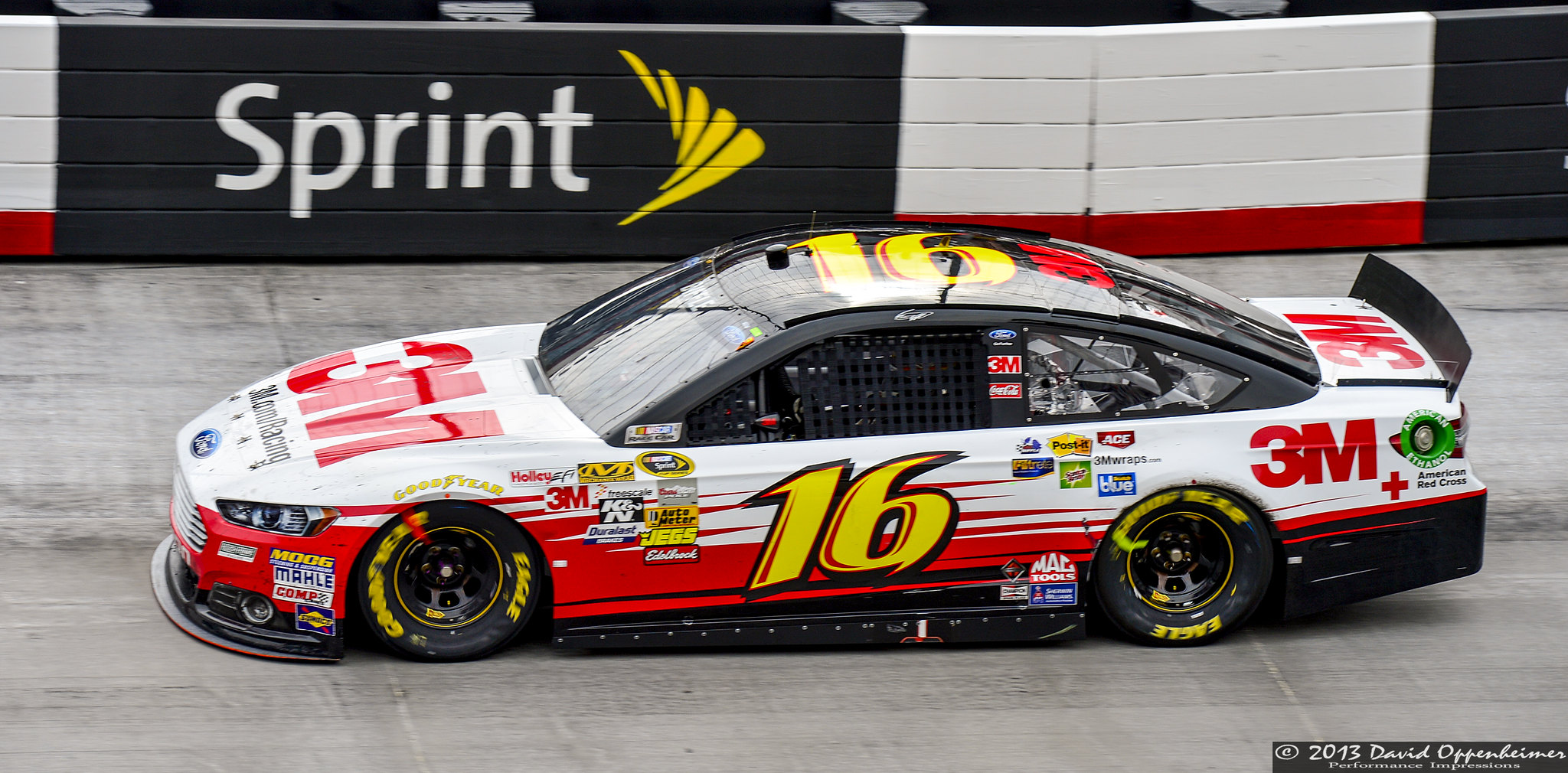This image captures a detailed view of a race car prominently displaying the number 16 in bold yellow on the top and side. The car, a sleek combination of white, red, and black, features "3M" in large red letters on the front hood and rear. Red and black spiky lines accentuate the sides, enhancing its dynamic appearance. The car is stationary on a gray track, likely during a NASCAR event, although no driver is visible. The background includes a segmented sidewall with a black rectangular Sprint advertisement featuring white letters and a yellow logo. In the bottom right corner of the image, the year "2013" and the name David Oppenheimer are visible, suggesting the photograph's attribution. The image is taken from a top angle, providing a clear view of the car’s profile and the surrounding track environment.